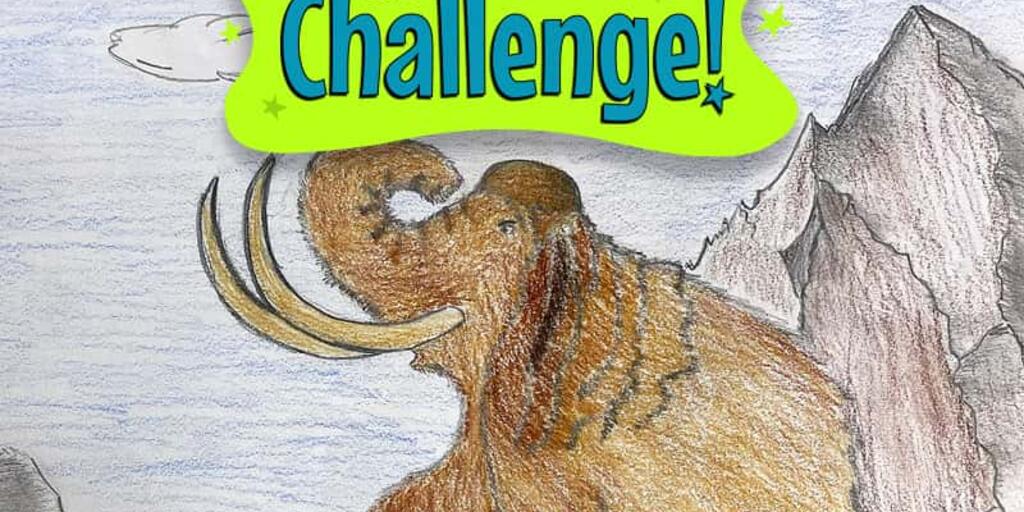The image showcases a detailed crayon drawing of a woolly mammoth with a distinct brown and reddish-brown fur. The mammoth's trunk is elegantly curled back over its head, and it features two pronounced, curved tusks extending forward. The mammoth appears to be wearing a form-fitting brown skull cap. Behind the mammoth, a rocky, peaked mountain is sketched, adding depth to the scene. The sky is colored light blue with a single white cloud positioned near the upper left. Dominating the top of the drawing is a bright green banner with the word “CHALLENGE” written in blue. Notably, where the dot of the exclamation mark would be, there is a star, mirrored by another lighter star at the opposite end of the banner. This lively and colorful artwork is reminiscent of a well-executed child’s drawing, possibly by a 3rd to 5th grader, showcasing careful attention to detail and vibrant use of color within the lines.